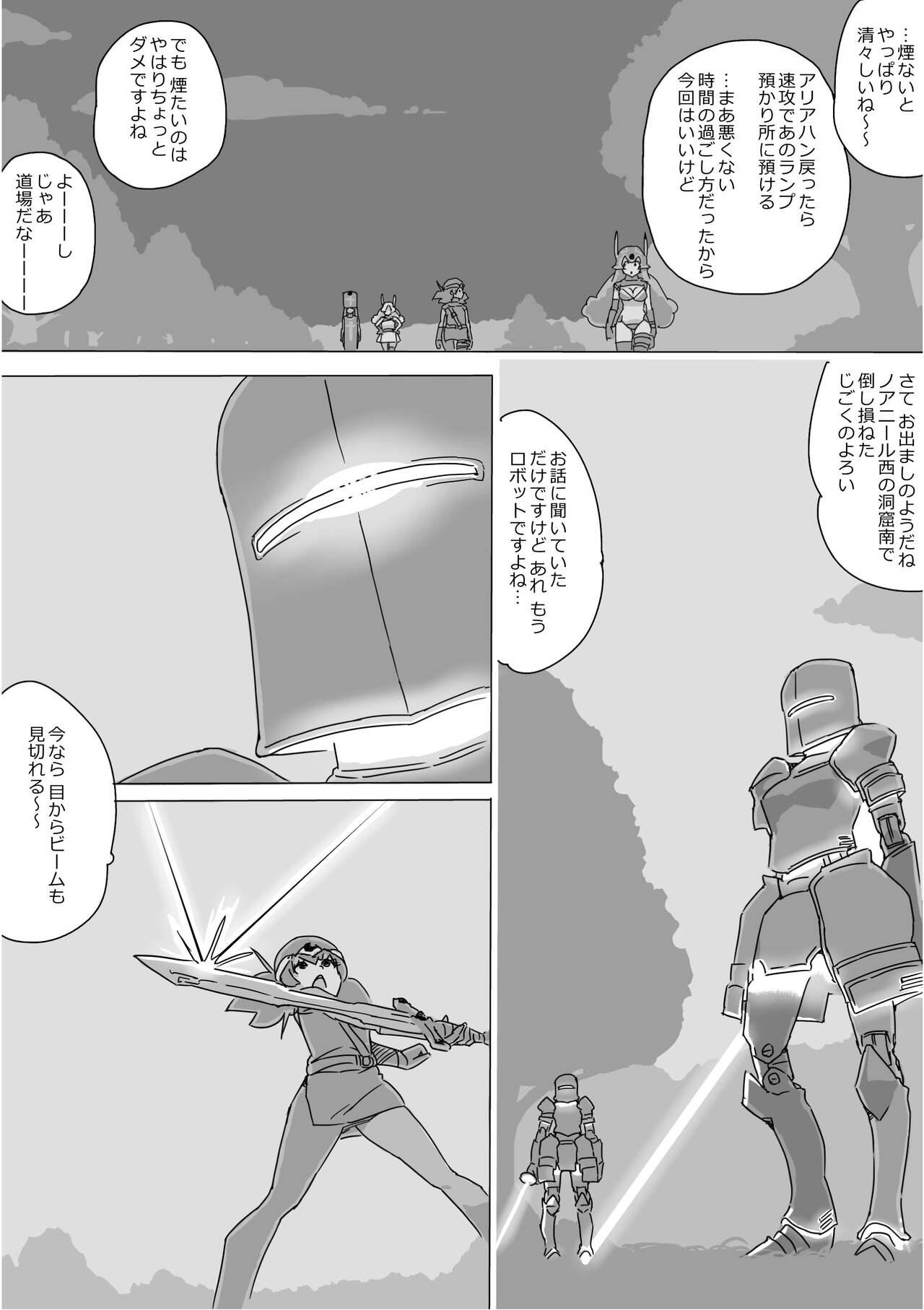This is a black and white comic strip featuring Japanese text. The layout consists of four panels, arranged in a detailed sequence.

- **Top Panel:** Spanning the entire width of the strip and occupying roughly the upper fifth of the image, this horizontal panel showcases a scene in a forest. It shows four characters walking, including a superhero-like figure with a cape leading the group. The figure on the right, distinguished by armor and long hair, suggests a commanding presence.

- **Right Vertical Panel:** Extending down the entire right side of the strip, this vertical panel depicts two armored, machine-like characters. One character is exceptionally tall, reaching the height of the trees, while the other is shorter. Both have shield-like faces and hold pristine white swords.

- **Left Vertical Panels:** Divided into two square-like sections stacked vertically, the upper panel presents a close-up of the tall machine character's masked face. The lower panel features a female character holding a sword, with the blade reflecting an unknown element, possibly deflecting a laser beam.

The entire comic strip is rendered in shades of gray and white, emphasizing the contrast between the characters and their surroundings.